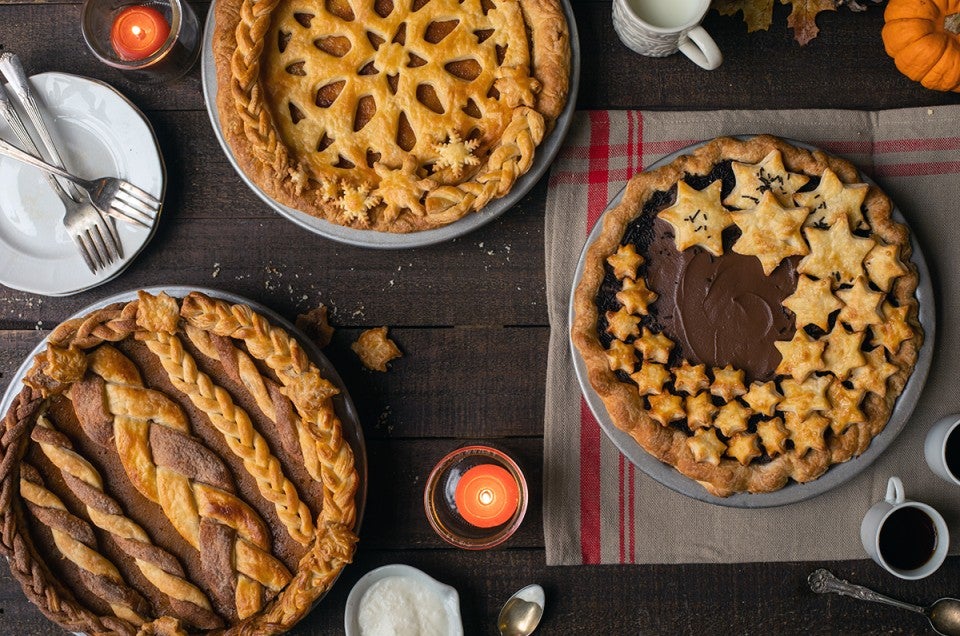A variety of beautifully crafted pies are displayed on a rustic wooden table. On the right side of the table, there are plates and forks neatly arranged, ready for serving. At the top of the image, a visually appealing pie features intricate details: a braided crust runs along one side, a large star cutout decorates the center, and smaller star cutouts are artfully scattered across the top. In the lower left corner, a pie with a rich chocolate or dark filling showcases a braided border and vertical braids of dough, adding an elegant texture. To the right, another chocolate-centered pie is adorned with a border of dough stars, creating a cohesive and charming circle of star-shaped decorations.